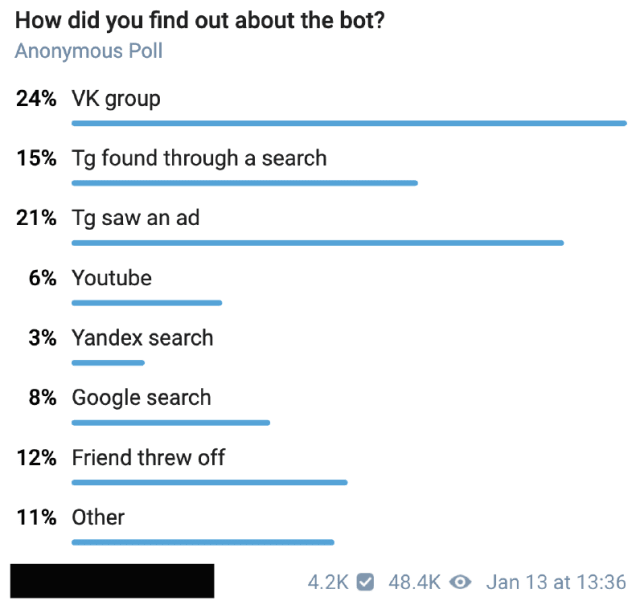This image is a screen capture displaying the results of an anonymous poll, featuring a clean, white background with various black, gray, and blue graphics. At the top, the question posed in bold black text reads, "How did you find out about the bot?" Beneath this, the subtext "anonymous poll" appears in gray.

The poll results are listed as follows:
- "VK group" at 24%, represented by a blue bar.
- "TJ found through a search" at 15%, with another blue bar.
- "TJ saw an ad" at 21%, also displayed with a blue bar.
- "YouTube" registers at 6%, shown with a blue bar.
- "Yadx search" has 3%, accompanied by a blue bar.
- "Google search" sits at 8%, marked by a blue bar.
- "Friend threw off" is at 12%, along with a blue bar.
- "Other" accounts for 11%, visualized by a blue bar.

Towards the lower portion of the image, there is an obscured black bar, which seems to blur or hide some information. Below this, in gray text, additional data is provided: "4.2 K" next to a gray box with a white check mark, "48.4 K" alongside an eyeball icon, and the timestamp "January 13 at 13:36." All poll percentages and source names such as "VK group" are rendered in black text, matched with corresponding blue bars.

The overall layout is described as user-friendly, with large, easily readable fonts, and a lack of pixelation or unnecessary blurring, ensuring clarity and accessibility.